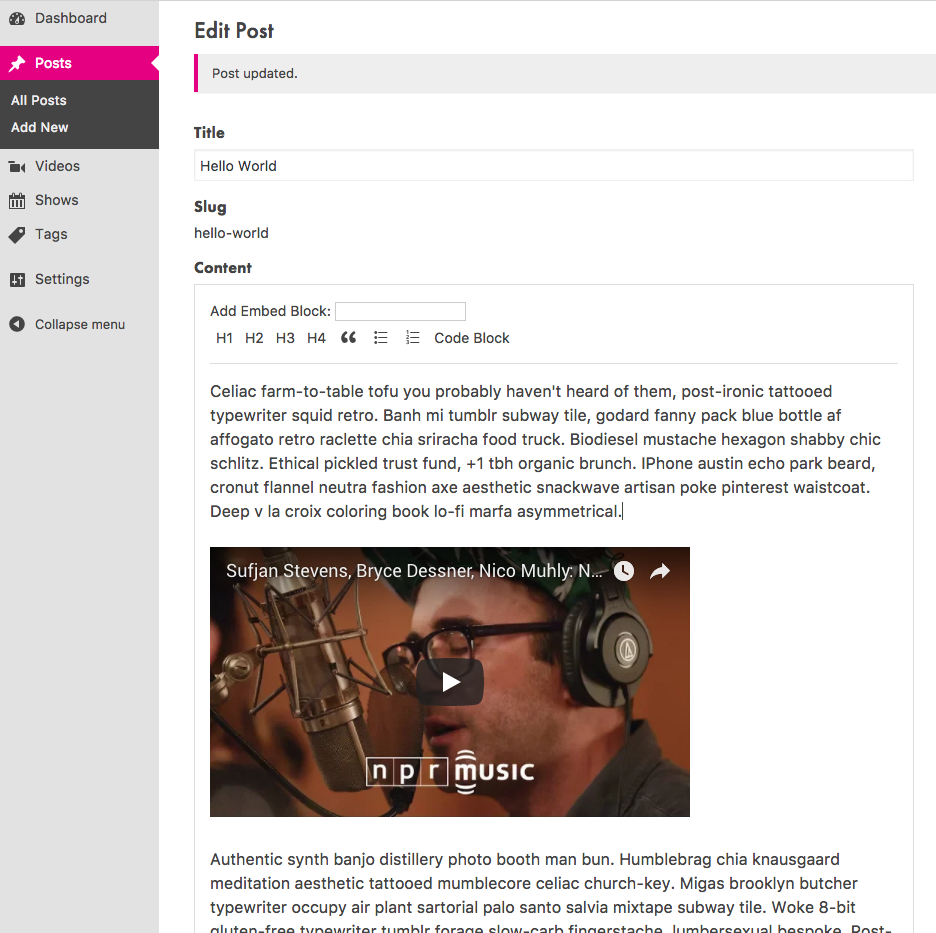In this screenshot from a media website, the interface is showcased with various features. On the left-hand side, there's a vertical gray sidebar that spans the length of the image. At the top left corner, several navigational tabs are visible, starting with "Dashboard" followed by "Posts," which is highlighted in pink and has a dropdown menu containing "All Posts" and "Add New." Below these, there are additional tabs labeled "Videos," "Shows," "Tags," and "Settings," along with an option to collapse the menu.

On the right side of the image, the background is predominantly white. At the top, the section is titled "Edit Post." Beneath this, a light gray notification bar indicates "Post Updated." The post title is "Hello World," and the slug is set as "hello-world." In the content area, there is an option to add an embed block. The visible content includes some text and a linked YouTube video featuring an artist in a recording studio, as depicted in the video thumbnail.